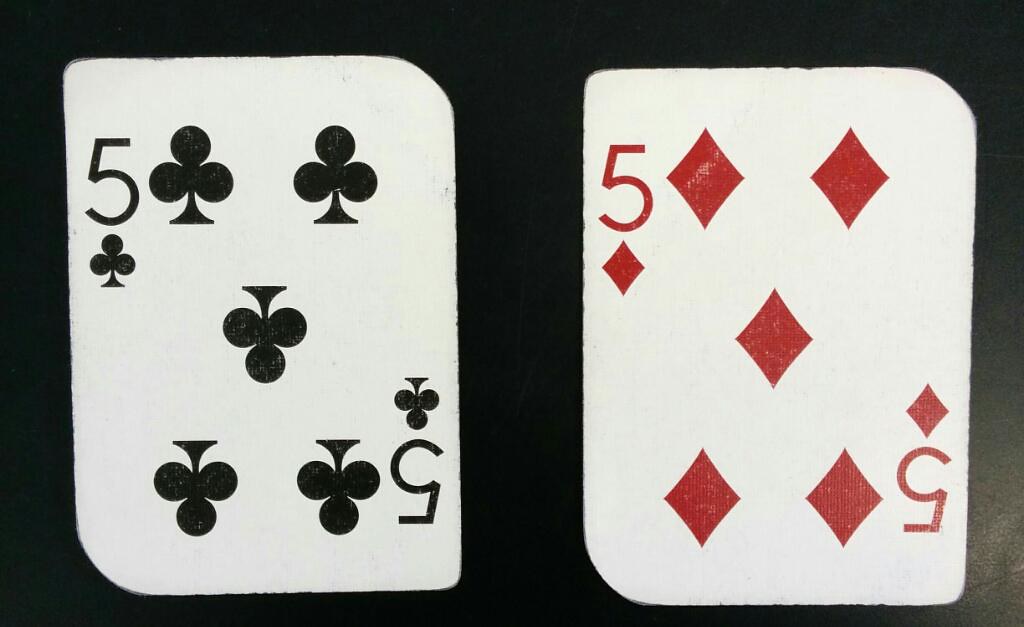The photograph features a simple yet striking composition against a black textured table surface. A subtle light source illuminates the lower right corner of the table, adding depth to the scene. Centrally positioned are two well-worn playing cards. The card on the left is the 5 of Clubs, identifiable by its crisp white background and black clover symbols, with a '5' marked at the top left and bottom right. To its right is the noticeably faded 5 of Diamonds, distinguished by its red diamond symbols and numbers, also placed in the upper left and lower right corners. Both cards reveal their age through rounded corners, dirt, stains, and ridged edges, indicating extensive use over time.